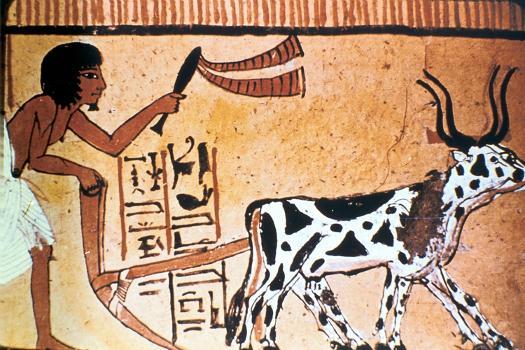This historical painting, resembling ancient Egyptian artwork believed to be found in temples or pyramids, vividly depicts a shirtless Egyptian figure with brown skin and very dark black hair. The man, adorned in a white garment and holding a whip-like instrument and a brown field tiller, is shown driving a cow forward. The cow is characterized by its white body adorned with black spots and prominent black horns. The background features hieroglyphics and pictographs, set against a light brown, sandstone-like wall. At the top of the image, a series of short brown vertical lines suggest the presence of a rooftop, bounded by a black horizontal line, contributing to the antiquated and almost caveman-like artistic style.